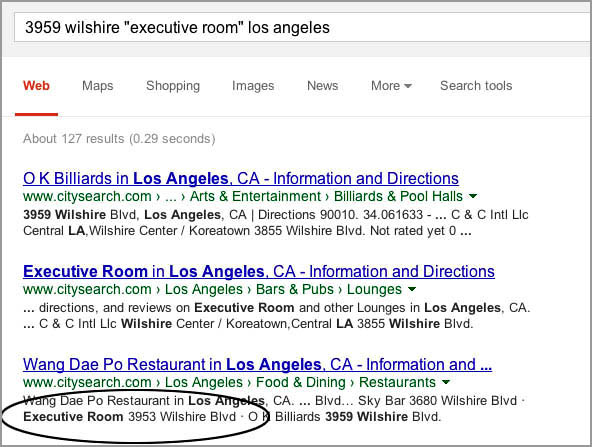The image features a data field displaying the address "3959 Wilshire Boulevard, Executive Room, Los Angeles." Below this information, options such as "Web," "Maps," "Shopping," "Images," "News," and "More" along with a dropdown menu and search tools are visible. Notably, "Web" is highlighted in red, while the other options are in gray with a red line underneath "Web." The results section shows approximately 127 results generated in 0.29 seconds.

Highlighted listings are present beneath this section. The first listing is "OK Billiards," located at 3959 Wilshire Boulevard, Los Angeles, categorized under arts and entertainment, billiards, and pool halls on Citysearch.com. The second listing is "Executive Room," also located at 3959 Wilshire Boulevard, Los Angeles, under the category of bars, pubs, and lounges on Citysearch Los Angeles. The third listing, encircled in black, is "Wang Dae Poe Restaurant," located at 3953 Wilshire Boulevard, Los Angeles, under food and dining, restaurants on Citysearch Los Angeles.

The color scheme of the image includes shades of white, gray, black, red, blue, and green, contributing to the overall visual presentation.